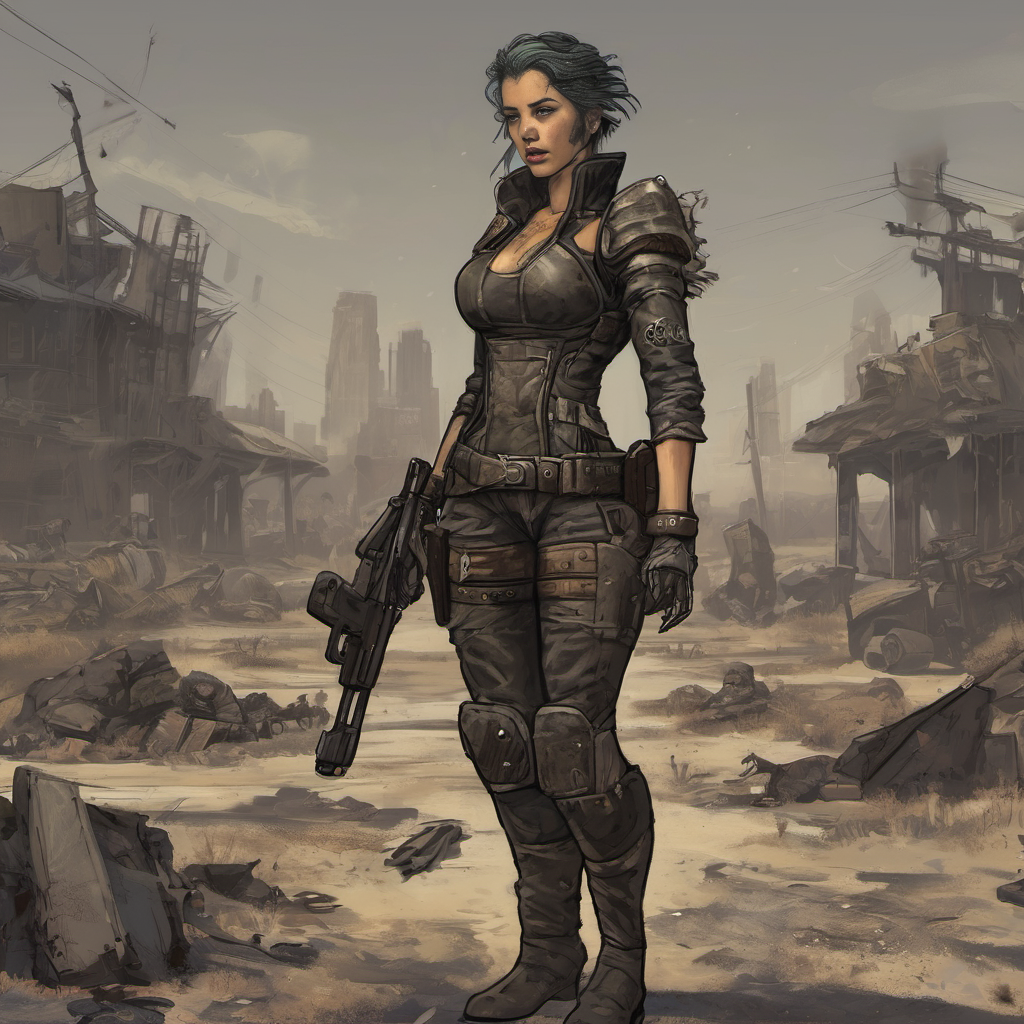A digitally created, square illustration-set within a post-apocalyptic, Wild West-inspired wasteland. The scene's backdrop is characterized by dilapidated wooden buildings, strewn debris, and a ground marked by various shades of creams and browns signifying recent destruction. The sky is partly visible, with some cloud coverage contributing to a hazy atmosphere, and a few taller buildings stand in the distance under this murky hue.

In the center stands a tall Caucasian woman, donned in a dark, paramilitary-style outfit. She has short, dark bluish-black hair that flows slightly behind her head. Her attire is detailed with black fatigues, a utility belt, and heavy-duty black pants tucked into high-heeled, tall boots. Her upper body is protected by metal shoulder pads, a chest plate with a low-cut collar, and elbow-length sleeves. Both knees are guarded by braces, accentuating her combat-ready appearance.

The woman is captured in a pose where she holds a machine gun in her right hand pointed downwards. Her left hand is gloved, adding to the rugged look. She gazes off into the distance with a stoic expression, embodying a resilient and solitary figure amidst the desolate ruins.